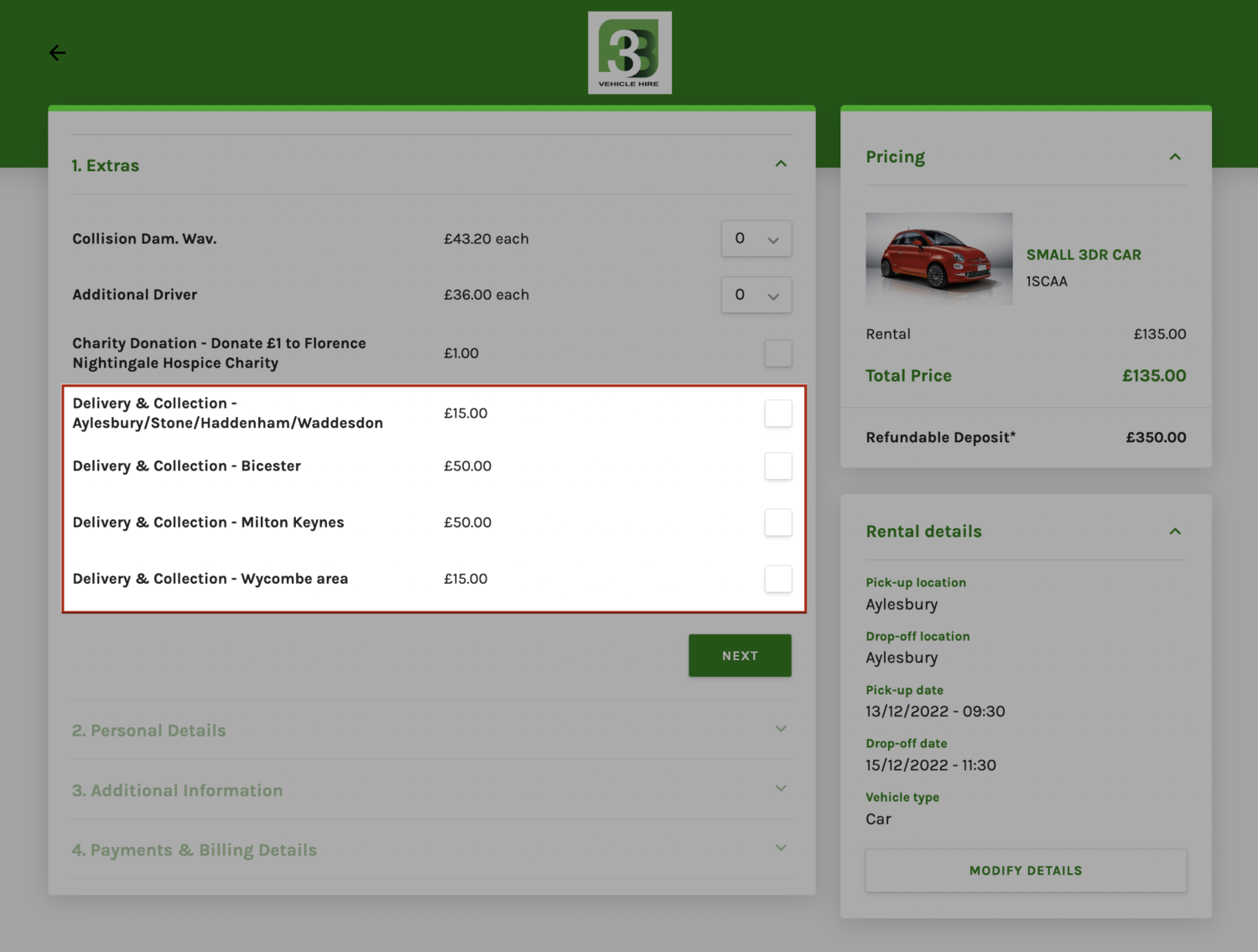The image depicts a webpage or user interface for a vehicle rental service. At the top of the page, there's a wide horizontal green rectangle. Towards the top left corner of this green segment, there is a black arrow pointing to the left. Centrally positioned within the green rectangle, the text "Vehicle Hire" is prominently displayed alongside a logo featuring the number '3' in white against a green background, with a black 'B' next to it.

On the left side of the page, there is a large black rectangle. Adjacent to this are two vertically stacked rectangles, each slightly larger than the left rectangle. The upper sections of these two stacked rectangles are highlighted in neon green.

Towards the center-right of the page, a bright white rectangle with a red outline stands out, containing black text that displays a price in pounds (£). Within this price box, there are four white checkboxes, all of which are unchecked.

Below the price rectangle, there's a green button labeled "Next" in white text. Further down, another box labeled "Pricing" includes an image of a red car. At the bottom, there is a section titled "Rental Details" featuring a button labeled "Modified Details" in green text.